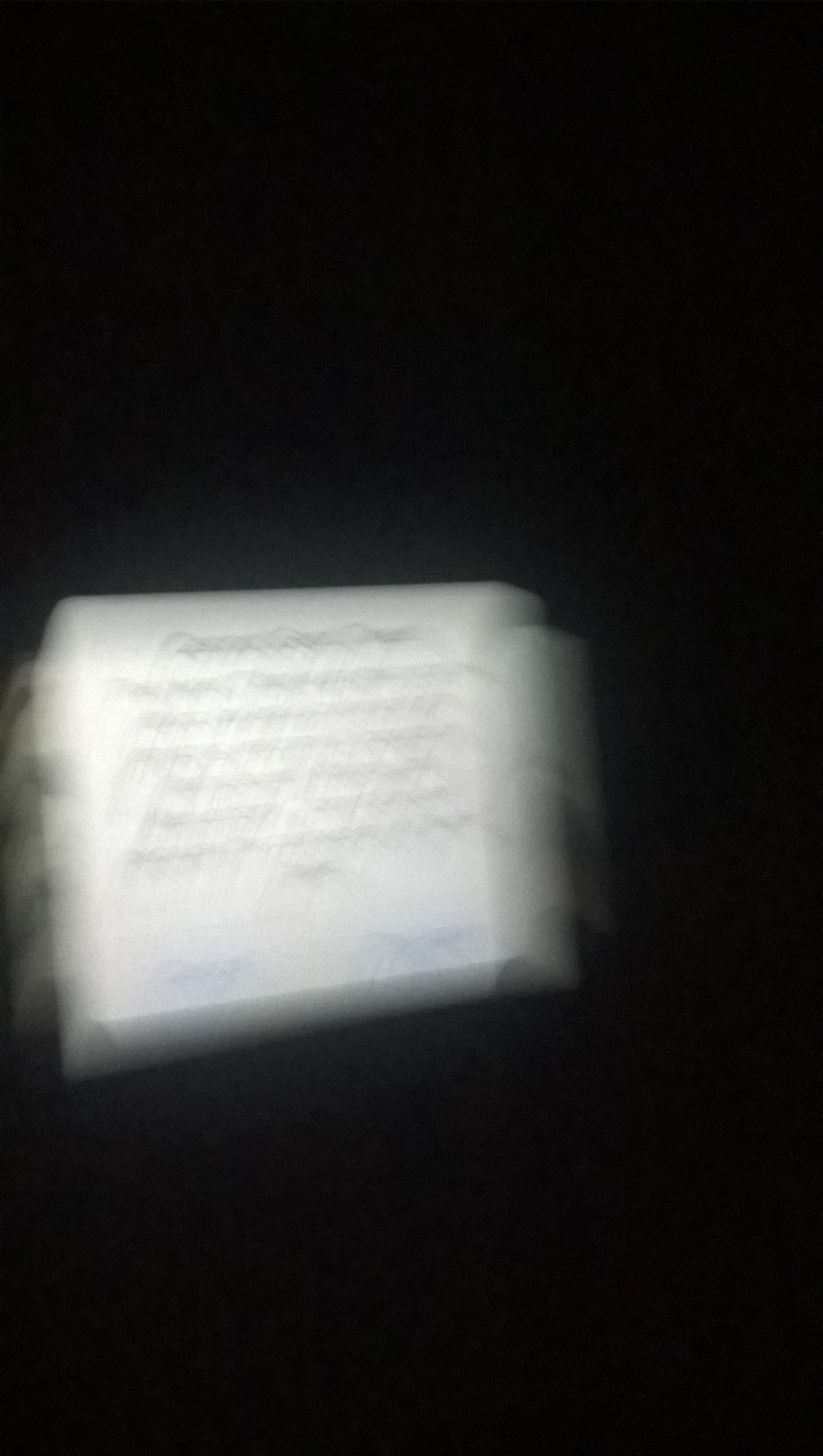In this image, the background is entirely black, which suggests either the room is dark or the wall behind is black. Positioned mid-left is a white piece of paper or possibly a screen displaying content. The photograph is extremely blurry, making the edges and the contents indistinct. Despite the blur, it is apparent that the displayed item contains a paragraph, a title, and two buttons at the bottom, though the text and details are impossible to discern due to the lack of clarity.